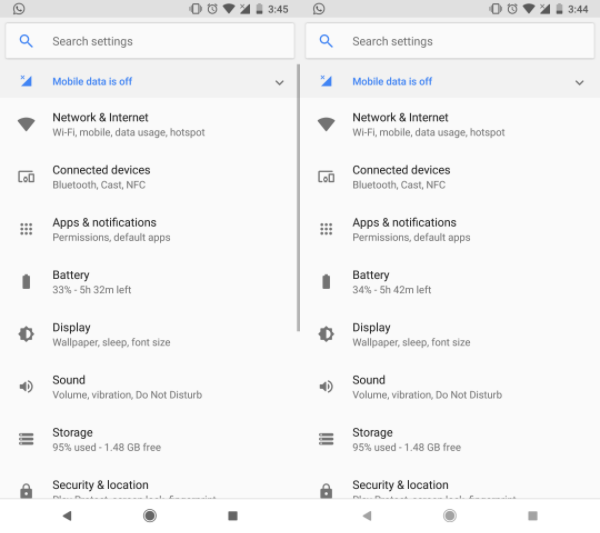The image displays two nearly identical screenshots taken from a mobile phone. Each screenshot is organized as vertical rectangles, with the respective times of 3:45 and 3:44 displayed in the upper right corners. At the top of both screenshots, the header reads "Search settings," accompanied by a search bar with a blue magnifying glass icon on the left side.

Both screenshots indicate that mobile data is turned off, shown in blue text near the top. Further down, the settings options listed are virtually identical on both screens:

1. **Network & Internet**
2. **Connected Devices**
3. **Apps & Notifications**
4. **Battery** (with a charge of 33% on the left and 34% on the right)
5. **Display**
6. **Sound**
7. **Storage**

The primary differences between the two screenshots are the battery percentages and minute discrepancy in the time displayed. The rest of the content is consistently the same across both images.